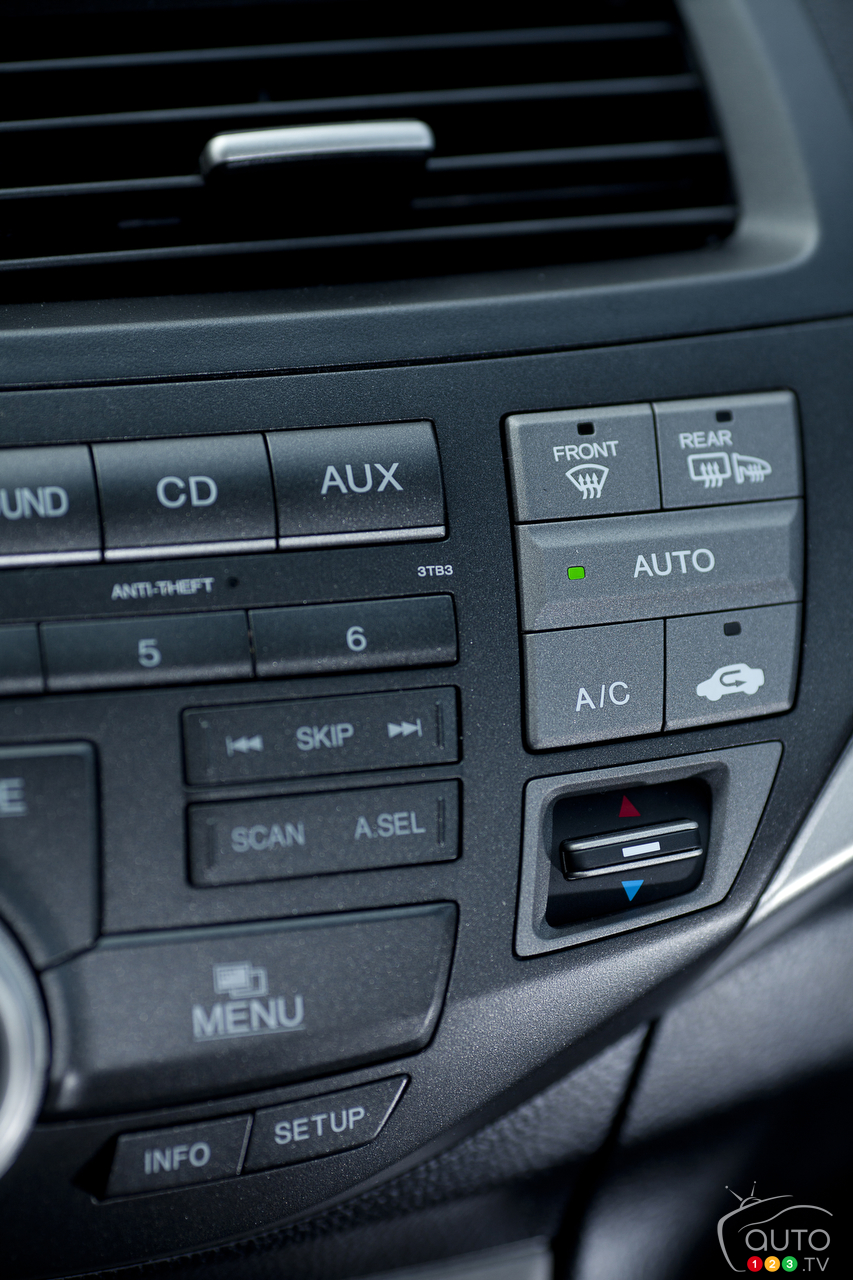This is a detailed close-up image of a car dashboard section. At the top, there is a vent with a silver knob, surrounded by predominantly black and gray controls that have a shimmery appearance under the light. Beneath the vent, you can see the controls for a CD player labeled "CD" and "AUX," next to "anti-theft 3TB3." Directly below are numbered buttons "5" and "6," followed by a "skip" button, a "scan" button, and a large "menu" button. Below the menu button, there are "info" and "setup" labels. 

To the right of these, there's another panel featuring lighter gray buttons with the labels "front" (showing a windshield icon) and "rear," indicating defrost functionality. Below that is an "AUTO" button illuminated with a green light, followed by "AC" and a button with an icon of a car and an arrow, indicating air circulation controls. At the bottom, there is a knob with a red arrow pointing up and a blue arrow pointing down, likely for temperature control. Finally, in the bottom right corner, there is the text "AUTO TV" and nearby red, yellow, and green circles. 

Overall, the dashboard is a mixture of various buttons and dials essential for controlling the car's functions.